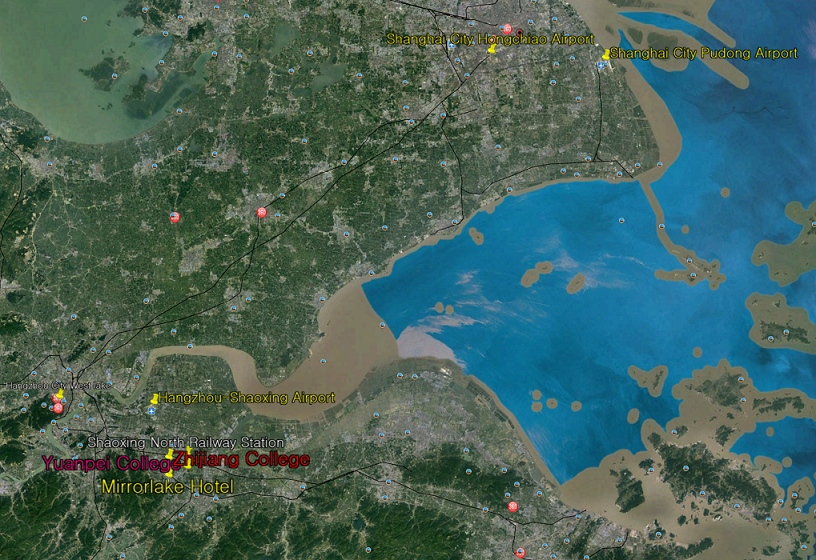This satellite image depicts a coastal region in China with numerous labeled locations and colorful pins denoting specific sites. The map features a mixture of terrain, with a significant water body extending from the center indentation towards the top right corner, dotted with small islands. Major landmarks include the Mirror Lake Hotel, Yuánpéi College, Zhejiang College, Shaoxing North Railway Station, Hangzhou Shaoxing Airport, and two prominent airports in Shanghai: Hongqiao and Pudong. Blue and red dots scatter across the map, indicating various points of interest, while the key locations are marked with yellow pins. Verdant greenery envelops much of the land area, especially on the left side, contrasted by the expansive water to the right.